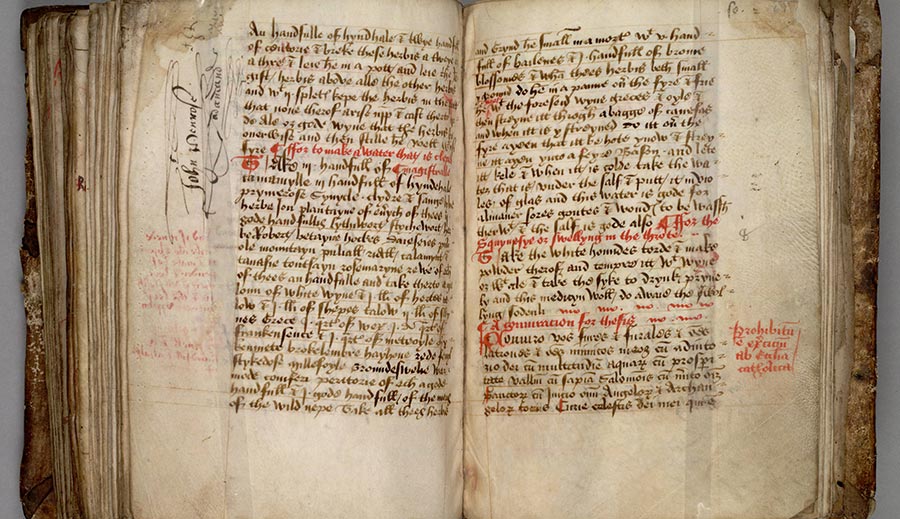The image showcases a close-up of an open illuminated manuscript, possibly dating back to the Middle Ages. The manuscript, bound in a worn and distressed cover, is displayed on a white tablecloth. The pages, tan and aged like parchment or vellum, are marked by ragged, creased, and deteriorated edges, with visible brown and red splotches. The text, written in a cursory or old-fashioned calligraphic font, appears to be in Latin, rendered predominantly in black ink with sections highlighted in red rubric ink. Some marginalia and additional text in red and black ink are visible alongside the main body of the script, some of which seem to be added notes or corrections. The top right and left sides of the book have tape or material and overlapping faded text. Overall, the manuscript exudes an aura of historical significance and delicate preservation.